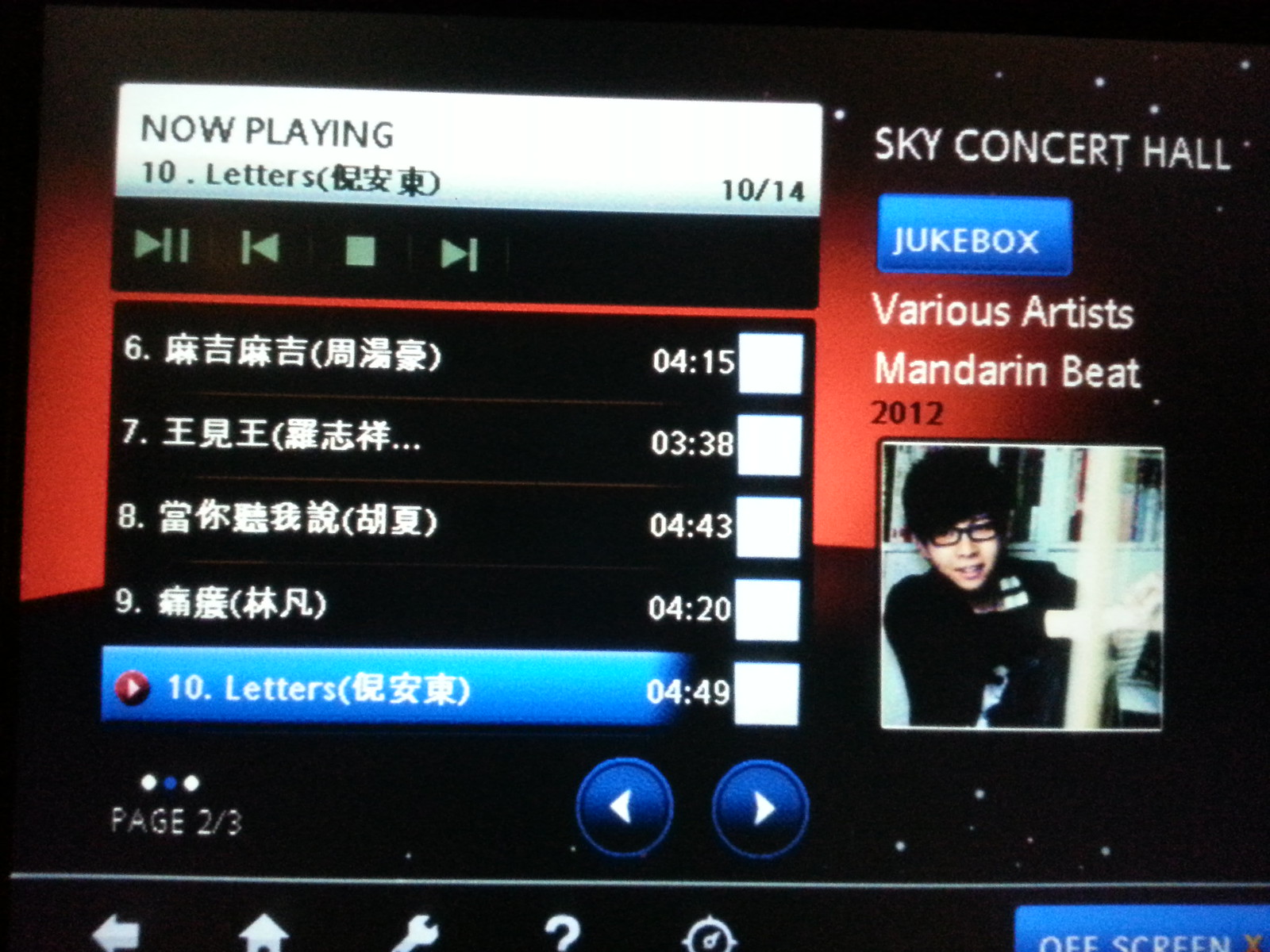In this image, we see a screenshot of a music app interface, which appears to be either on a computer or a mobile phone. The screen is primarily in Chinese, except for a few English words. On the left side, there's a numbered list of songs, currently displaying a section from 6 to 10. The song "Now Playing" is listed as number 10, titled "Letters," accompanied by a duration label indicating it's the 10th track out of 14 total songs. Below this track are other songs, each with their respective durations. Central to the bottom of the screen are playback controls including fast forward, rewind, pause, and play buttons, facilitating navigation through the playlist. To the right, the app features a label "Sky Concert Hall" followed by a blue button labeled "Jukebox." Below this is the text "Various Artists, Mandarin Beats 2012." Accompanying this text is an image of a young man, presumably a Chinese singer, with long black hair and glasses, wearing a black shirt, likely representing an album cover. The bottom left corner indicates "Page 2 of 3," suggesting multiple pages of song listings.